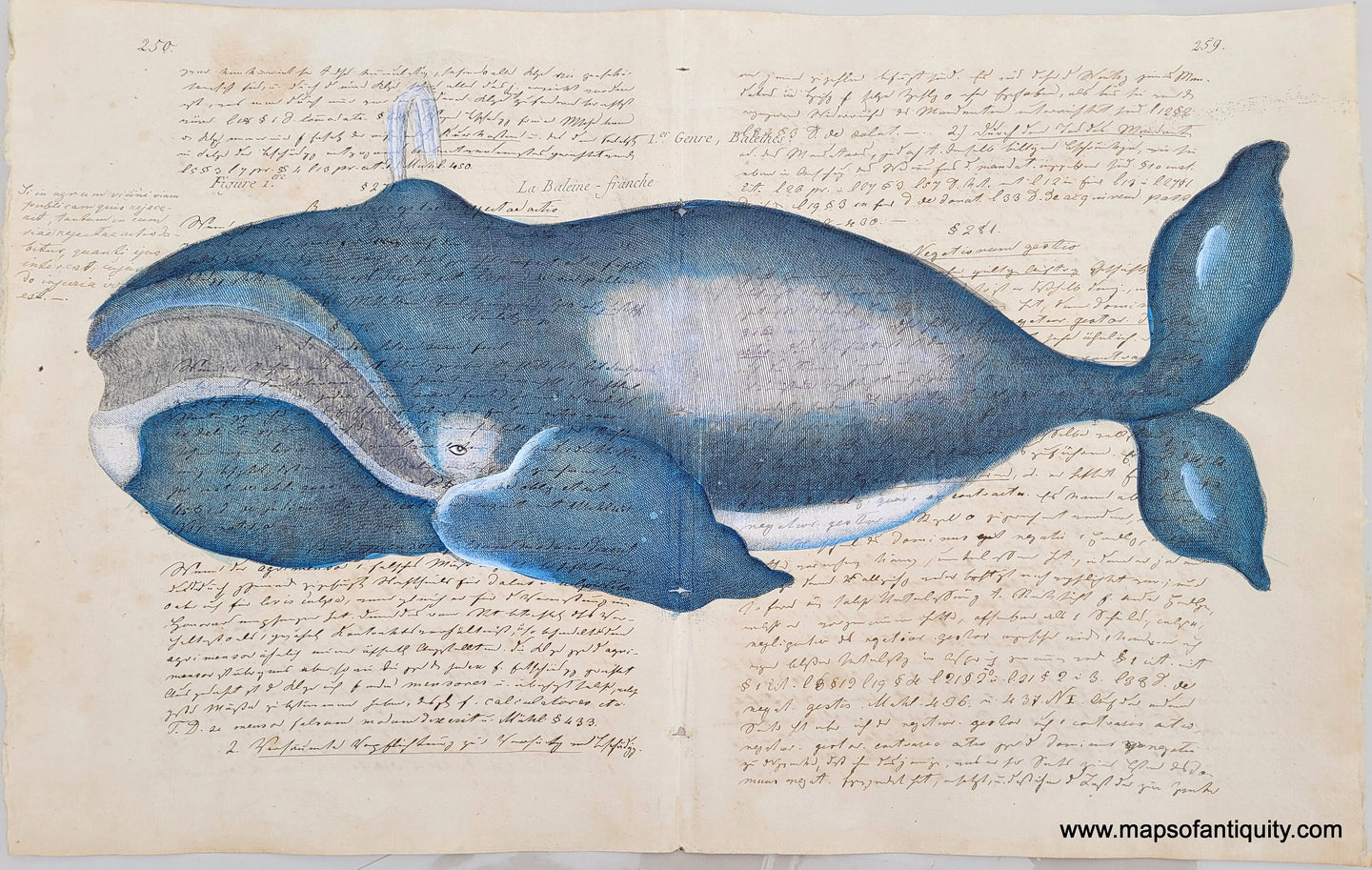The image depicts a digital scan of an extremely old, handwritten manuscript, likely resembling a diary or historical data, open to display both the left and right pages. The top left page is marked as 258 and the top right as 259, with the text densely filling both pages in faint, cursive black ink. A large, bluish whale illustration spans across the center of the text, its head on the left page and its tail extending onto the right. The whale is light blue with white areas around its belly, midsection, eyes, and a gray mouth, depicted as if shooting water from its blowhole. Despite the whale's playful expression, its presence obscures more than half of the handwritten content. The bottom right corner of the image bears a watermark from www.mapsofantiquity.com, and the text, though mostly unreadable, is clearly antiquated and possibly in another language.